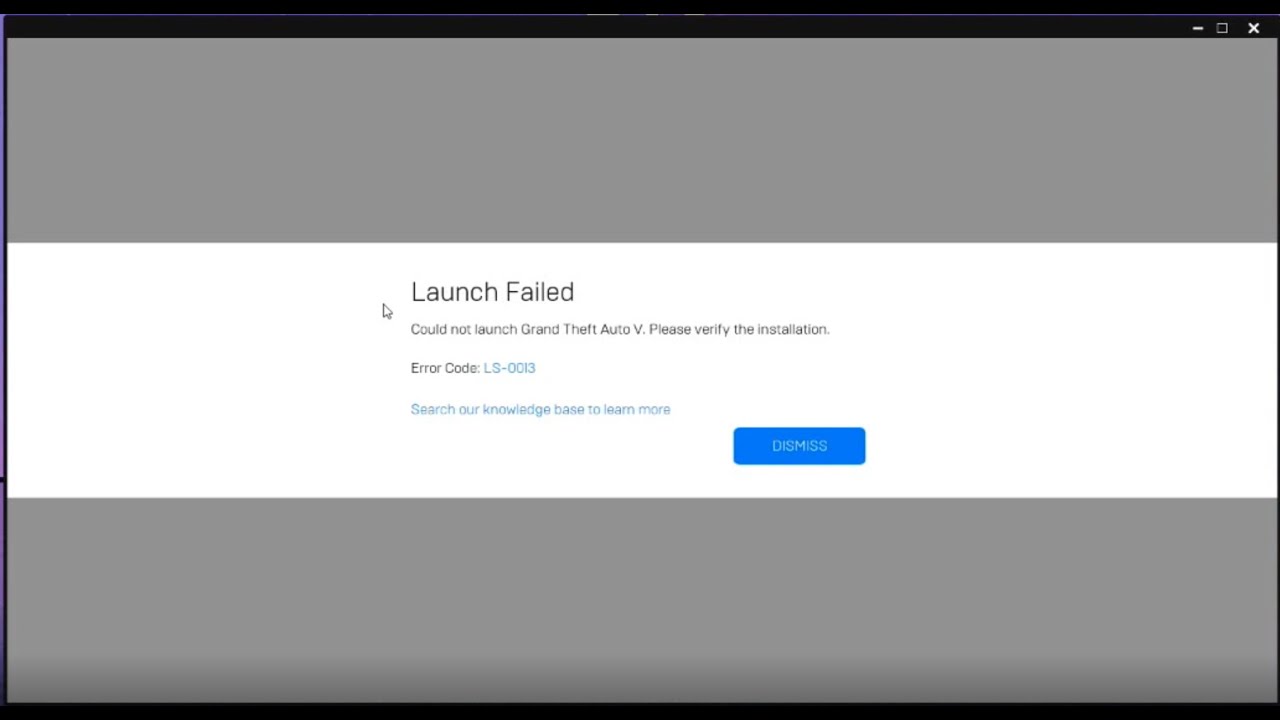### Descriptive Caption:

This image displays a screenshot from a computer screen, showcasing a game launcher interface for Grand Theft Auto V. The interface is framed with a black border resembling the outline of a computer monitor. In the top-right corner are the standard window control buttons: minimize, window resize, and close (X).

The screen is divided into three horizontal sections. Both the top and bottom sections are a slate gray color, effectively empty. The middle section stands out with a white background, where most of the information is located.

At the top left of this white section, in black text, are the words "Launch Failed. Do not launch Grand Theft Auto V." Underneath that, a line of blue text reads "Error code: LS-0013." Below that, another blue text line offers assistance with "Search our knowledge base to learn more."

Towards the bottom-right of the screen, there is a prominent blue button with white text that says "Dismiss." A mouse cursor is visible, indicating user interaction.

Overall, the screenshot captures a failed game launch attempt, with instructions and an error code provided, and the option to dismiss the alert.